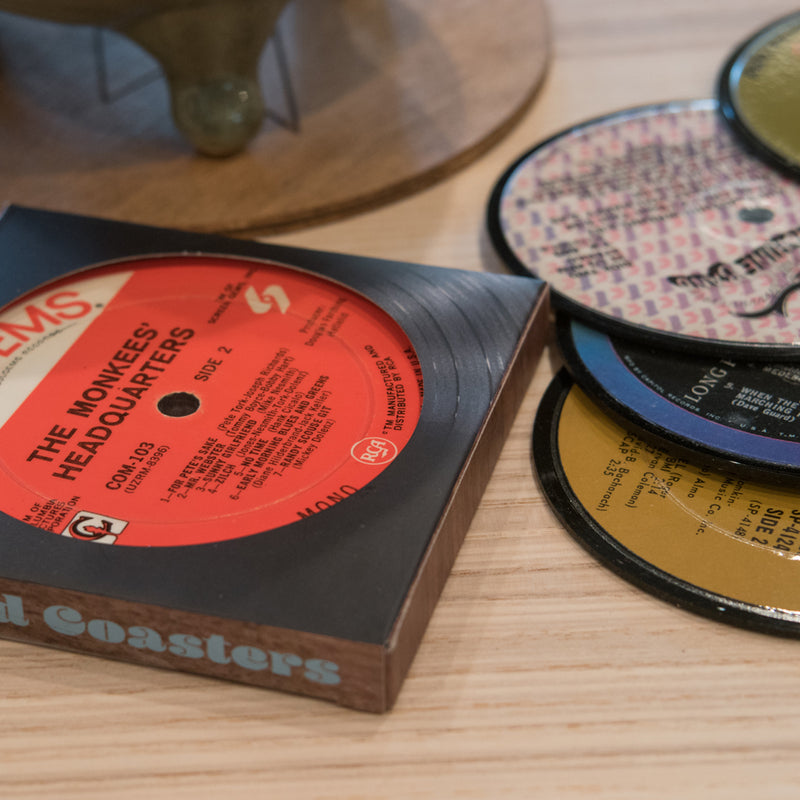The image depicts a set of vinyl-themed coasters arranged on a light wood surface. The central coaster mimics a red CD with black capital letters reading "THE MONKEES HEADQUARTERS" and a track listing below it. It prominently features the text "SIDE TWO" to the right of the center hole and "COM-103" with additional serial number information to the left. This coaster is bordered by a raised vinyl-like print square. The word "COASTERS" appears in light blue on the spine of the coaster's box, nearest to the camera's perspective.

To the right, four other coasters are partially visible, each designed to look like different colored CDs. The top-right coaster is dark green, the one below it has a mix of purple and pinkish-orange shapes, the next one down is blue with a black center, featuring white text, and the bottom-most coaster is brown with a slight yellow tinge, also covered in black text. These coasters are stacked in a scattered manner, with their designs adding to the vinyl record theme.